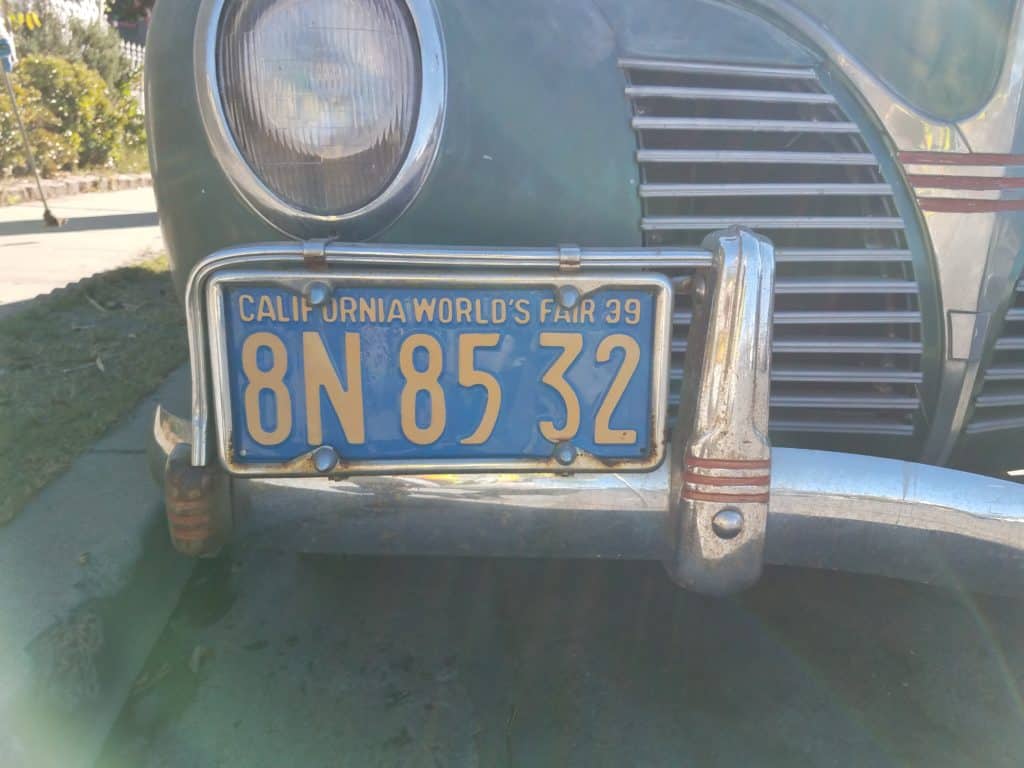This color photograph captures a close-up view of the front end of an old automobile, specifically focusing on the license plate and surrounding details. The vehicle, which seems to date back to the late 1930s, is light blue in color and features a unique license plate reading "California World's Fair 39" with the alphanumeric code "8N 8532," all inscribed in yellow against a blue background. This plate is mounted slightly off-center, towards the passenger side, and is secured with stainless steel brackets and screws. Just above the plate, the car's oval-shaped headlight, outlined in silver, is visibly prominent. The silver grille of the car adds additional vintage charm to the image. The automobile is parked on a cement surface with a curb and a patch of grass beside it. The background features a white picket fence and trees, with sunlight reflecting off the cement walkway, adding a nostalgic glow to the scene.